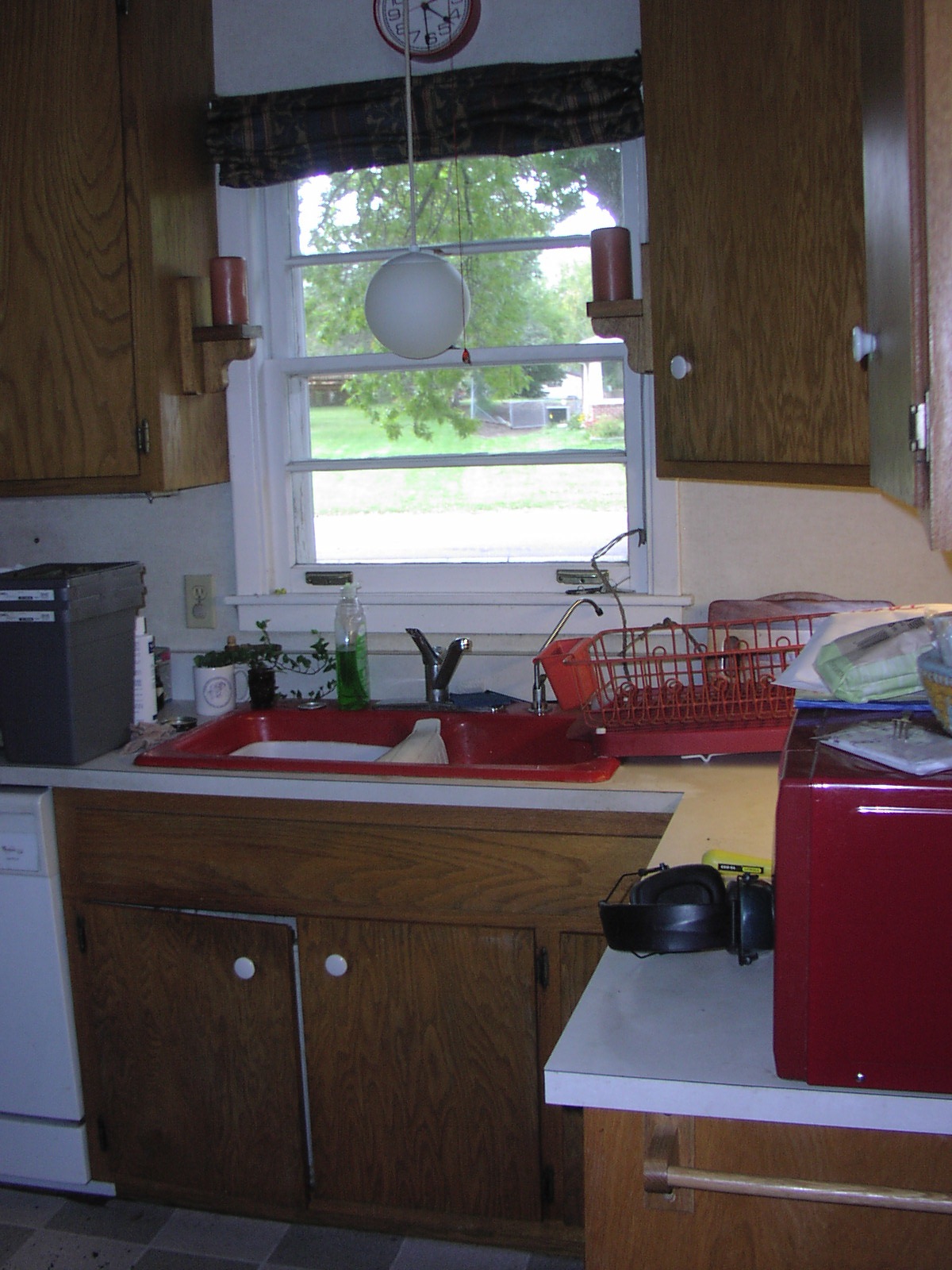The image depicts a retro-style kitchen, likely from the 1990s. In the bottom left corner, there's a white dishwasher with a black note or writing on it. The surrounding cabinetry is crafted from brown wood with white knobs. The sink, which is vivid red with a silver faucet that can be lifted to release water, is designed as a dual-basin. The left basin contains a white bin. 

To the left of the sink, there's a clear, ovoid-shaped bottle of green dish soap along with a metallic red dish rack. In front of the sink, a pair of bulky headphones rests against a rectangular electronic device, likely a microwave, though only its left side is visible. Adjacent to the left of the sink stands a white mug adorned with a blue circle, containing something blue whose details are unclear. 

A small black flower pot with green leaves sits nearby, adding a touch of nature to the scene. Lastly, a white electrical outlet can be seen next to the white windowsill located behind the red sink.